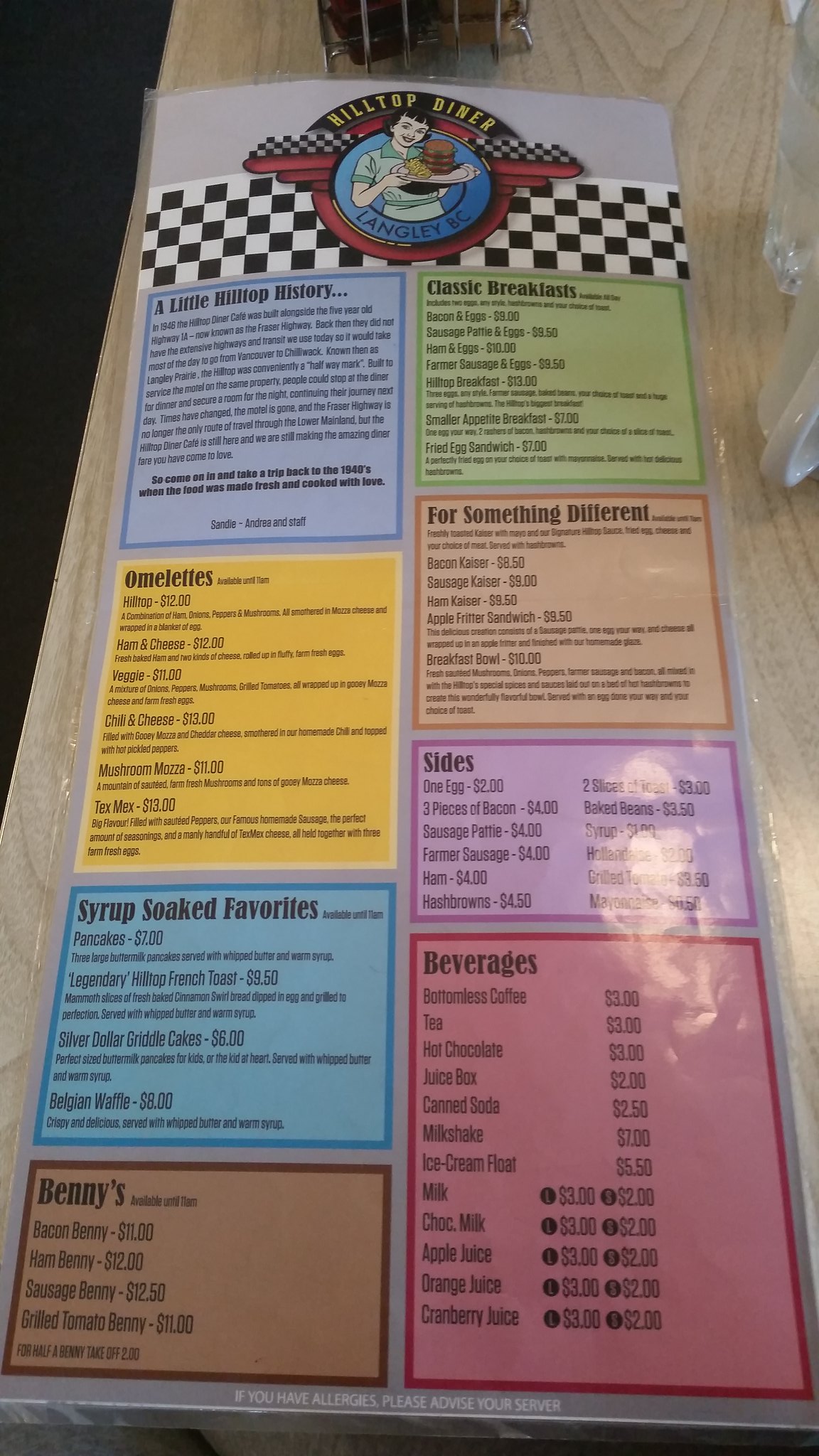A detailed photograph of a colorful, vintage-style menu sits prominently on what appears to be the counter of a restaurant. Above the menu, partially cut off, there is a syrup dispenser and to the right, a glass of water and the handle of a classic diner-style coffee cup are visible, hinting at the bustling atmosphere of the establishment. 

The menu is divided into a series of vividly colored squares and rectangles, each section featuring different offerings. At the very top, the restaurant's logo catches the eye with a charming checkerboard pattern. Superimposed on the checkerboard is an illustration of a cheerful waitress holding a burger, accompanied by the text "Hilltop Diner, Langley, BC."

- The upper left section, highlighted in a purplish hue, shares a piece of "Hilltop History," likely recounting the diner's storied past.
- Adjacent to it, a bright yellow block lists a variety of omelets.
- Below, a lighter blue section titled "Syrup-Soaked Favorites" features breakfast staples like pancakes and waffles.
- Directly beneath the blue section, in a warm brown, the menu showcases specialties called "Benny's," including options like sausage Benny and bacon Benny.
- On the upper right, a green rectangle displays "Classic Breakfasts."
- Directly below the green, a lighter brown section encourages patrons to try "For Something Different," where items like a breakfast bowl are listed.
- Another purple section below this offers various "Sides," mentioning items such as three pieces of bacon or ham.
- Finally, the bottom right, shaded in red, lists a range of beverages from milk and hot chocolate to tea and coffee.

The colorful sections and varied textures in the menu design reinforce the lively, inviting ambiance of Hilltop Diner, making it clear why it’s a cherished spot in Langley, BC.